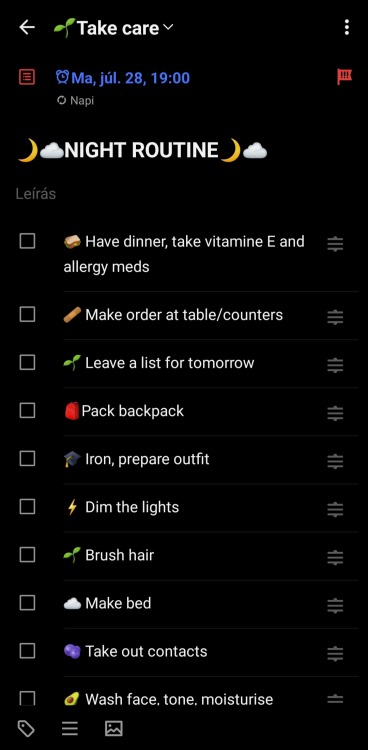In this image, we see a smartphone screenshot displayed in portrait mode, featuring a lifestyle or scheduling application. The top section of the screen prominently displays a title that reads "Take Care," indicating a caregiving or self-care schedule. Following this title is a date notation that appears to be "J-U-L" with an accent above the "U," suggesting the month of July in Spanish.

The primary language used within the app seems to be English, despite the Spanish date notation. Below the date, there is a label titled "Night Routine," outlining a comprehensive list of tasks to be completed as part of an evening regimen. The detailed list of tasks includes:

1. Have dinner
2. Take vitamin E and allergy medications
3. Organize the order at table counters
4. Leave a list of tasks for the next day
5. Pack the backpack
6. Iron clothes
7. Prepare the outfit for the next day
8. Dim the lights
9. Brush hair
10. Make the bed
11. Take out contacts
12. Wash face
13. Apply toner and moisturizer

This extensive list provides a thorough guide for a structured and organized night routine.